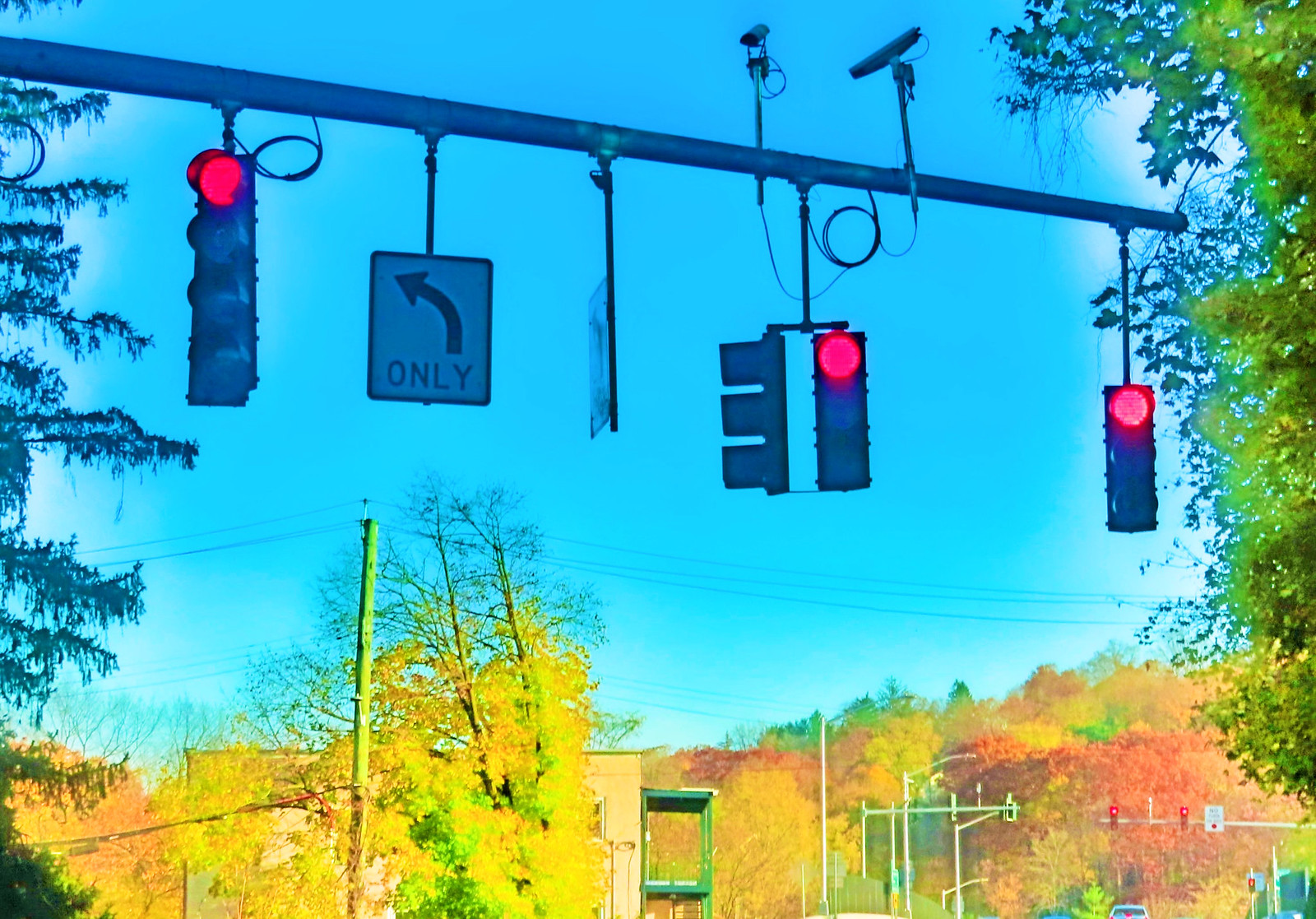The image depicts a bustling outdoor urban scene centered around a prominent intersection. A series of traffic lights are affixed to a sturdy metal pole; the three main traffic signals display glowing red lights. A fourth signal, oriented to the left, has its lights turned away from the viewer. Notably, the leftmost traffic signal contains four individual lights, while the others feature only three. A directional sign attached to the pole exhibits an arrow curving to the left with the word "ONLY" printed prominently. Above the signs and signals, two security cameras are positioned, likely monitoring the intersection.

The colors in the image seem somewhat altered, possibly through photo editing software, making everything appear overly saturated. The trees are especially vivid, with exaggerated shades of yellow, green, orange, and red. On the left side of the frame, part of a tree is visible. The sky is a striking bright blue with a few white clouds along the edges, adding to the surreal color palette. In the background, additional street lights, poles, and power lines can be seen, along with a building featuring a green terrace along its side. The overall composition captures the energetic atmosphere of the city, with a peculiar emphasis on vivid, saturated colors.